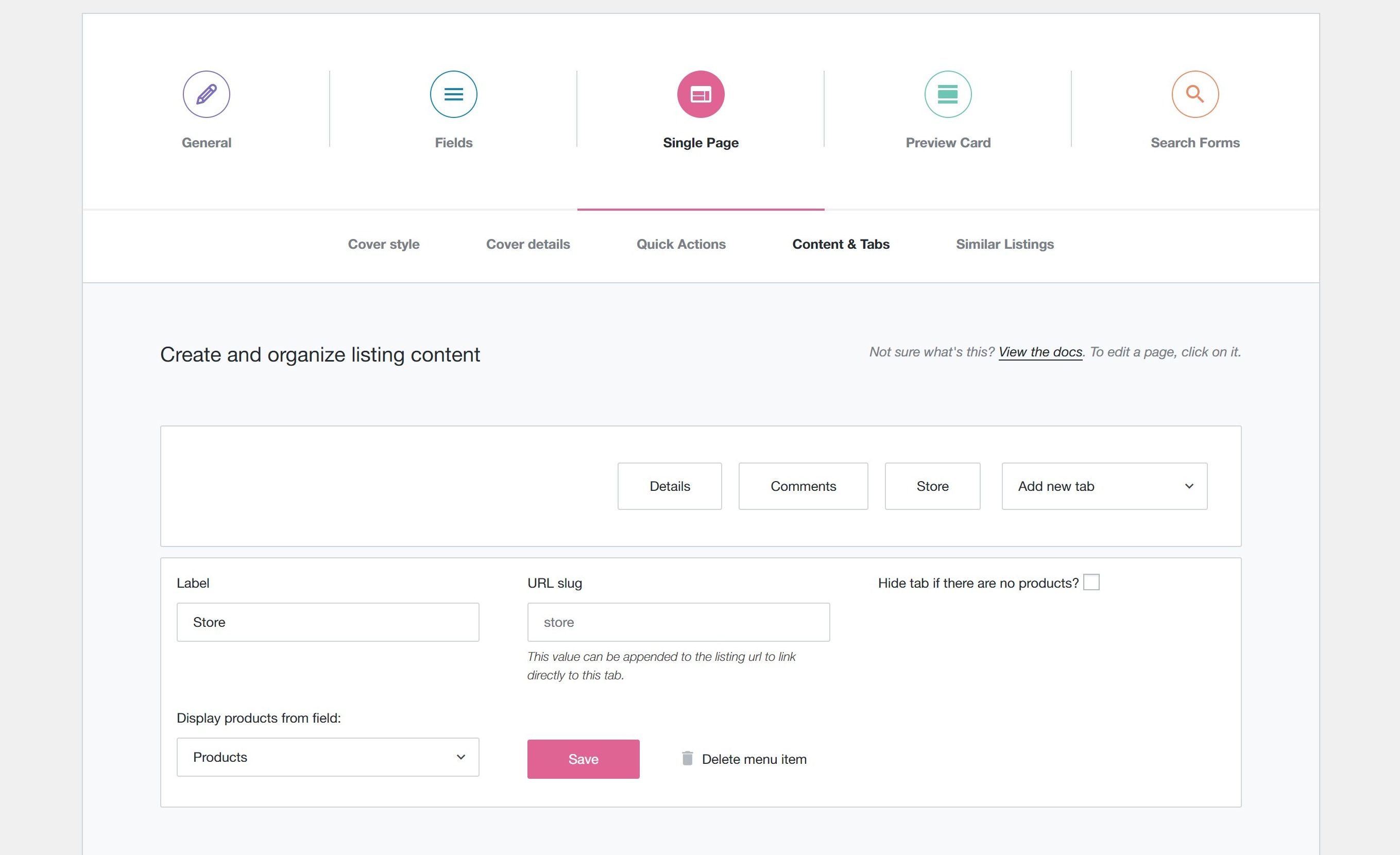In this image, we see a detailed interface of a website featuring various sections and icons, each with distinct colors and labels. 

At the top left corner, there's a light purple circle with a pencil icon, accompanied by the label "General". To its right, another circle with a greenish hue and a "hamburger" menu icon is labeled "Filled". 

Continuing to the right, the next section is denoted by a pink circle with a calendar-like icon and the label "Single Page". Further right, there are labels for "Preview Card" and "Search Forms". 

Below this horizontal menu, in the bottom middle, there are five categories listed: "Cover Style", "Cover Details", "Quick Actions", "Content and Tabs", and "Similar Listings".

The main content area underneath features a large greyish background. At its top left, the text reads "Create and organize listing content". On the far right, a prompt says "Not sure what's this? View the docs. To edit a page, click on it." 

In this section below the introductory text, there are two boxes. The first box includes options for "Details", "Comments", "Store", and "Add New Tab". The second box displays fields for "Label", "Display Products From", "Field", and "URL Slug". 

Additionally, there is a prominent "Save" button with white text on a pink background.